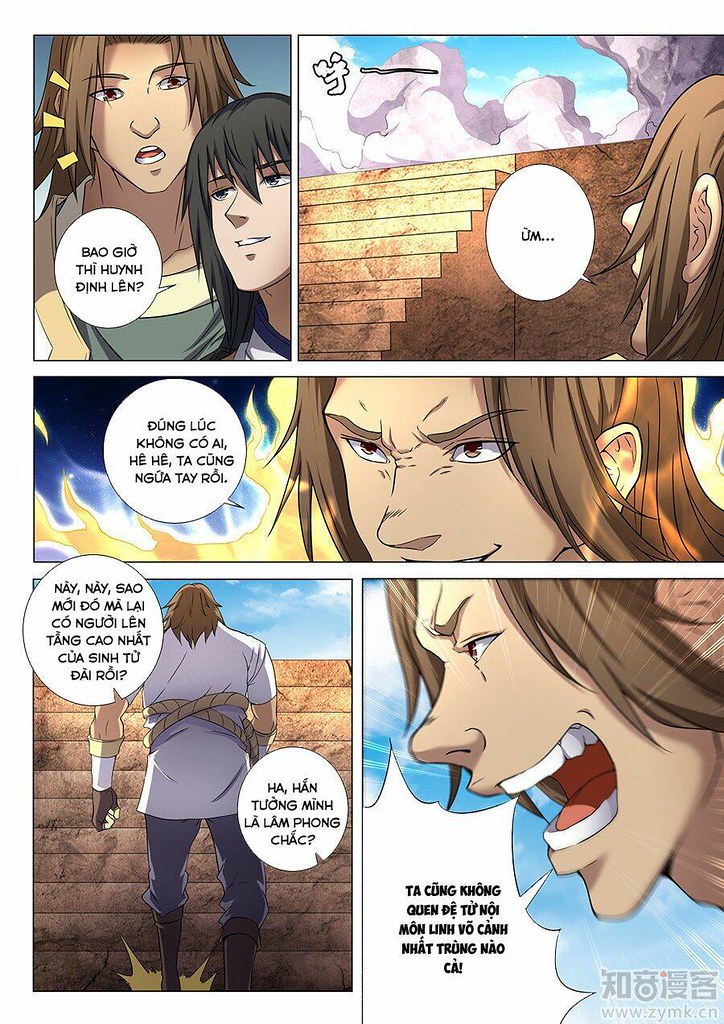This cartoon strip, likely from a comic book, consists of five detailed sections. The top left panel features two animated male characters, one with long brown hair and the other with dark, spiky hair who appears to be speaking in an unreadable language. In the top-right panel, the brown-haired individual is seen in front of flames or fire, possibly saying "um" as they look around. Surrounding them are steps leading up and clouds or smoke in the sky. The middle section focuses again on the brown-haired person. In the bottom left panel, we see the back of the brown-haired person, now appearing large and dressed in a white shirt and blue jeans, with descriptive words encircling them. The final bottom-right panel depicts the brown-haired character yelling, with their bolded text emphasizing their outcry, all within white speech bubbles written in a different language.